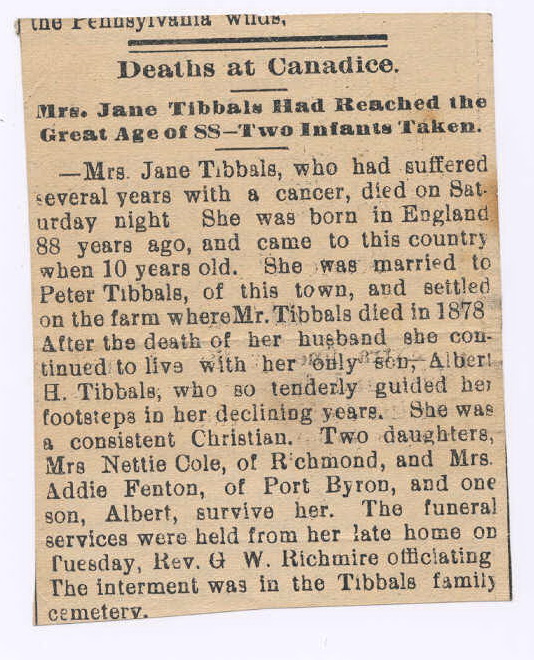This photograph captures a vintage, faded newspaper clipping presented against a white background. The aged paper exhibits notable creases, wrinkles, and small stains. The print is slightly ghosted by the text on the reverse side. At the top of the clipping, there are a few horizontal lines below which the headline reads, "Deaths at Canadice." Below this, the text states, "Mrs. Jane Tibbles had reached the great age of 88, two infants taken." The article describes Mrs. Jane Tibbles, who had suffered from cancer and passed away on a Saturday night. Born in England 88 years ago, she immigrated to the United States at the age of 10. She married Peter Tibbles and lived on their farm until his death in 1878. Mrs. Tibbles continued to reside on this farm with their only son, Albert H. Tibbles, who cared for her in her later years. She was remembered as a dedicated Christian. Survived by two daughters, Mrs. Nettie Cole of Richmond and Mrs. Addie Fenton of Port Byron, and her son Albert, Mrs. Tibbles' funeral services were conducted at her home with Reverend G.W. Richmire officiating. She was interred in the Tibbles family cemetery.